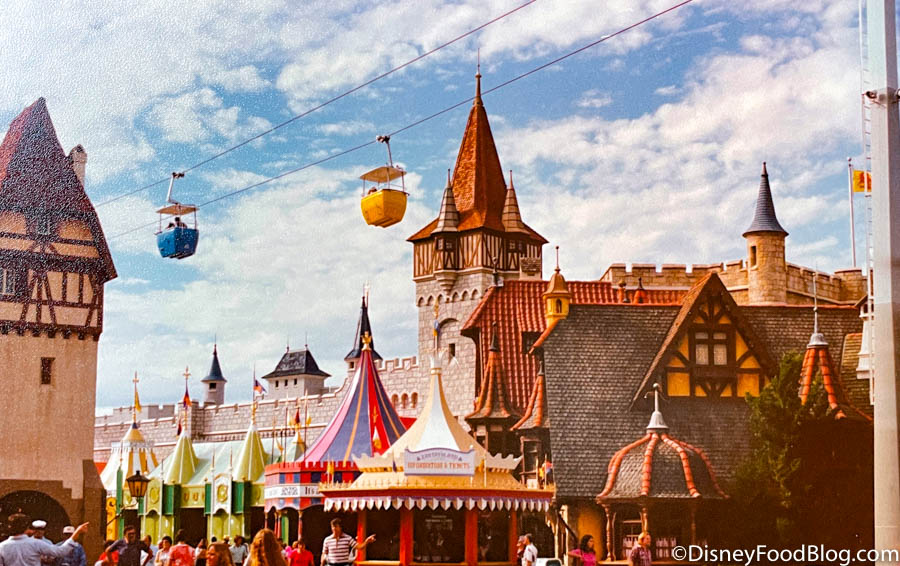This image, likely computer-generated or painted, captures an amusement park scene reminiscent of a vintage or medieval-themed area within Disney. The foreground is filled with people milling about, pointing, and talking, adding a lively atmosphere. A myriad of colorful buildings and tents with steep, spiral roofs in vibrant shades of green, blue, red, yellow, and white dot the landscape, resembling structures for food stands, ticket kiosks, and possibly carousels. Notably, a prominent man in a white and blue striped shirt stands near one of these structures, pointing towards it.

The backdrop features a grand castle with iconic steep spiral roofs and accompanying castle walls, hinting at a fairytale aesthetic. The scene above is punctuated by a sky ride with cable cars of blue and yellow, floating against a backdrop of a bright blue sky filled with fluffy white clouds. Close to this, there are two prominent high towers, possibly part of the larger castle structure, contributing to the medieval ambiance.

The entire image exudes a sense of festivity and elaborate architectural design, blending both artificial and traditional materials. At the bottom right, the copyright text "DisneyFoodBlog.com" marks the image's authenticity and possible origins from Disney's Magic Kingdom. The overall scene portrays a bustling, picturesque town full of color, life, and whimsical charm.